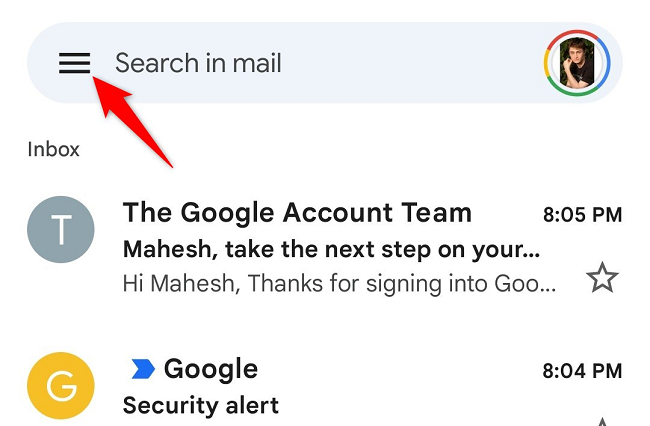In the image, we are presented with the interface of an email inbox. At the top left, there is a prominent search bar in the "Mail" tab, highlighted by a red arrow pointing towards a three-line menu icon. To the right, the familiar Google circle symbol can be seen, containing a profile image of a person inside.

Directly below the search bar, the "Inbox" label is displayed, indicating there are two items within. The first item features a blue circle with a white "T" inside, followed by the sender's name, "Google Account Team," and the time stamp, "8:05 PM." The email subject reads, "Mahesh, take the next step on your...", which is followed by a brief preview, "Hi, Mahesh. Thanks for signing into Google." Part of the word "Google" is cut off, showing only "G-O-O". Additionally, there is a star symbol next to this preview.

The second item in the inbox shows a gold circle with a white "G" inside, next to which is a blue arrow pointing towards the word "Google," written in black letters. The subject of this email is "Security alert," with the corresponding time stamp listed as "8:04 PM."